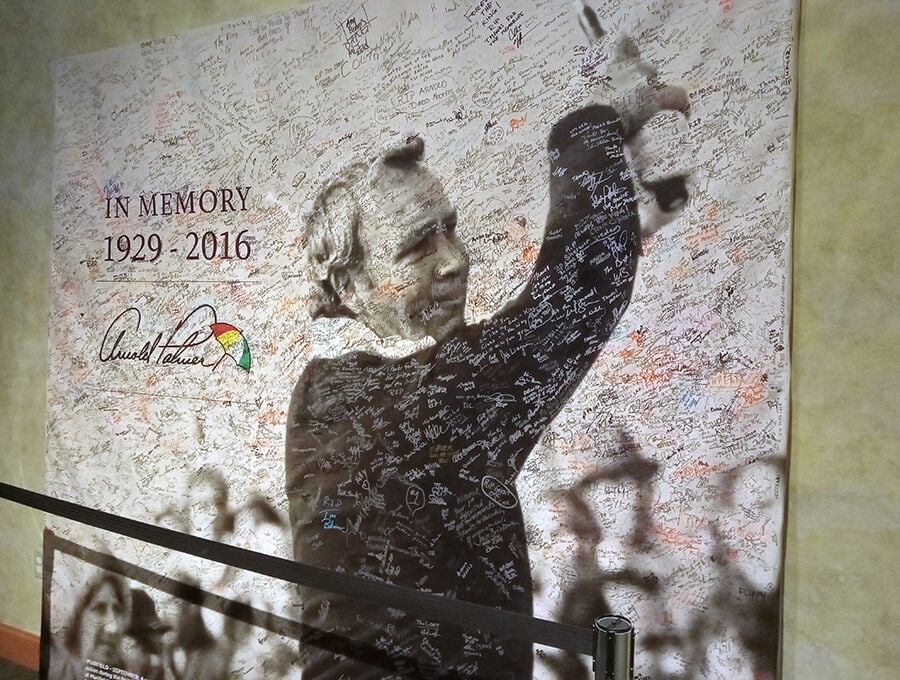This detailed image depicts a large commemorative poster honoring the legendary golfer Arnold Palmer, who lived from 1929 to 2016. The central figure in the poster is Arnold Palmer himself, seen from behind, yet his profile is clearly visible as he holds a golf club high in the air, as if acknowledging the crowd or following through on a swing. He is dressed in a black sweater over a white collared shirt, embodying his iconic style. The image of Palmer is set against a blurred backdrop of spectators, capturing the many fans who celebrated his illustrious career. Covering nearly every inch of the poster, from Palmer's shirt to the background of spectators, are countless heartfelt messages and signatures left by fans and admirers, demonstrating the profound impact he had on many lives. To the left is the poignant text, "In memory, Arnold Palmer, 1929-2016," along with his signature in cursive and a colorful umbrella symbol featuring red, yellow, white, and green stripes. The entire poster, appearing to be mounted against a wall, is cordoned off by a small roped area supported by metal poles, marking it as a significant memorial site.